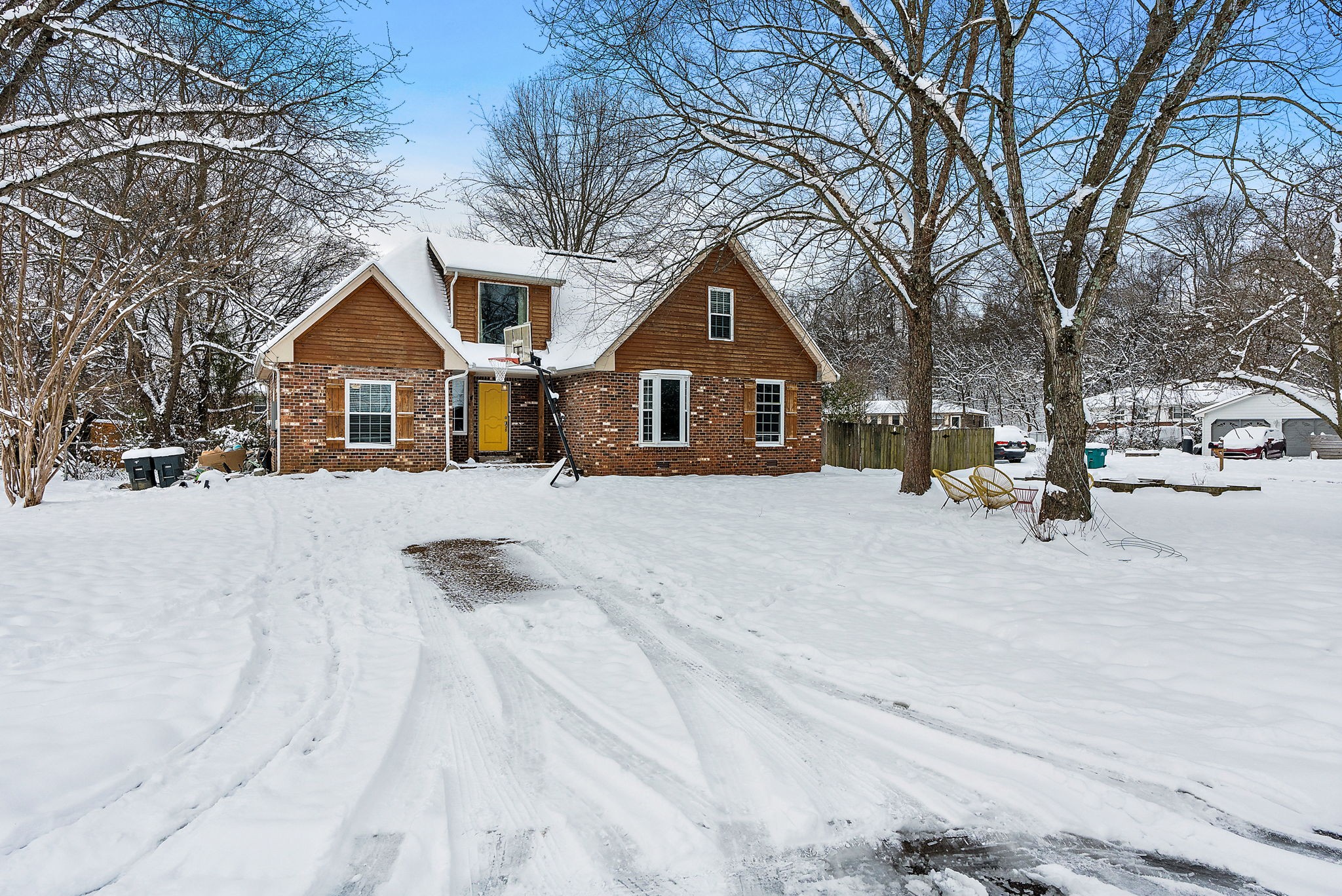This image captures the wintry, picturesque facade of a house. The scene is covered in a blanket of snow, no more than six inches deep, spreading across the ground and the roof of the house. Dominating the center of the image is a two-story home with a distinctive design: the first floor made of red brick and the second floor adorned with medium-colored horizontal wood planks. The house features a bright yellow door and windows outlined in white, adding a vibrant contrast to the winter landscape.

Surrounding the house, on both sides, are clusters of bare trees, their branches dusted with snow. Particularly on the left, several snow-covered trees are visible, while two additional bare trees stand prominently in front of the house on the right. A bright blue sky with puffy clouds near the bottom forms the idyllic backdrop, enhancing the serene atmosphere.

On the right side, the image captures additional elements: a white outbuilding with gray doors that appears to be a garage, and in the background, another white, snow-covered structure seemingly another house. In front of the main house, a field of snow is visible with a noticeable patch showing some pavement and tire tracks, suggesting recent vehicular movement. Near the trees, one can spot some wicker chairs, adding a subtle touch of rustic charm to the overall scene.